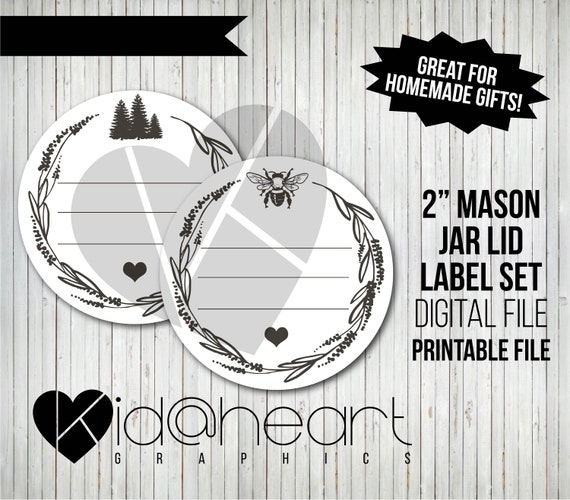This is an advertisement created by "Kid at Heart Graphics," featuring a 2-inch mason jar lid label set available as a digital, printable file. The ad, rendered in a rustic, gray, black, and white color scheme, prominently showcases two circular mason jar lid designs in the center, slightly off-set towards the top left. One lid features a bee graphic, while the other displays trees, each adorned with a small heart at the bottom. Text bubbles scattered around highlight key points: "Great for homemade gifts" is situated in the top right corner, and to the right of the lids, the text reads "2-inch mason jar lid label set, digital file, printable file." The overall aesthetic combines a rough cottage style with budget-friendly clip art elements, making it ideal for personalizing homemade jams, jellies, or creative DIY projects involving mason jars.